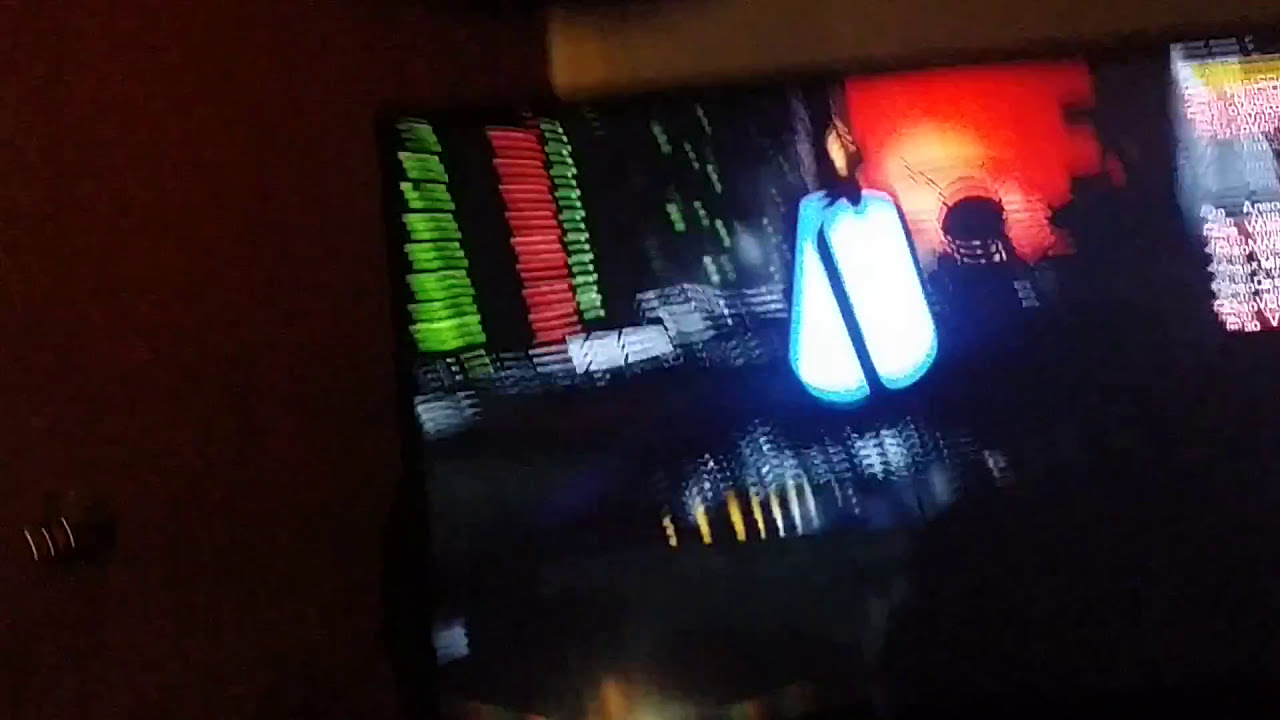This is a wide rectangular photograph capturing the inside of a dark room with several illuminated monitors lined up side-by-side on a reflective desk. The image is very blurry, suggesting it was taken in motion. The left side of the room is predominantly dark with hues of black and slightly dark brown.

Just left of the center, there is a screen displaying several rows of neon green text over a black background. Adjacent to it is another screen with a similar setup, but with glowing red text. Below these monitors, there's a keypad emitting white light. On the right side of the image, another screen features unreadable white text with red shadows, and it fades into yellow at the top. Further to the right, a larger screen displays a captivating sunset, where the sky is tinged red and the sun glows bright yellow.

Dominating the middle of the scene is a somewhat cone-shaped, bright neon blue light, which seems to float above the desk, illuminating the surrounding area. This unique light, coupled with the colors from the monitors, casts various reflections on the desk’s surface, creating an atmospheric and somewhat mysterious ambiance.